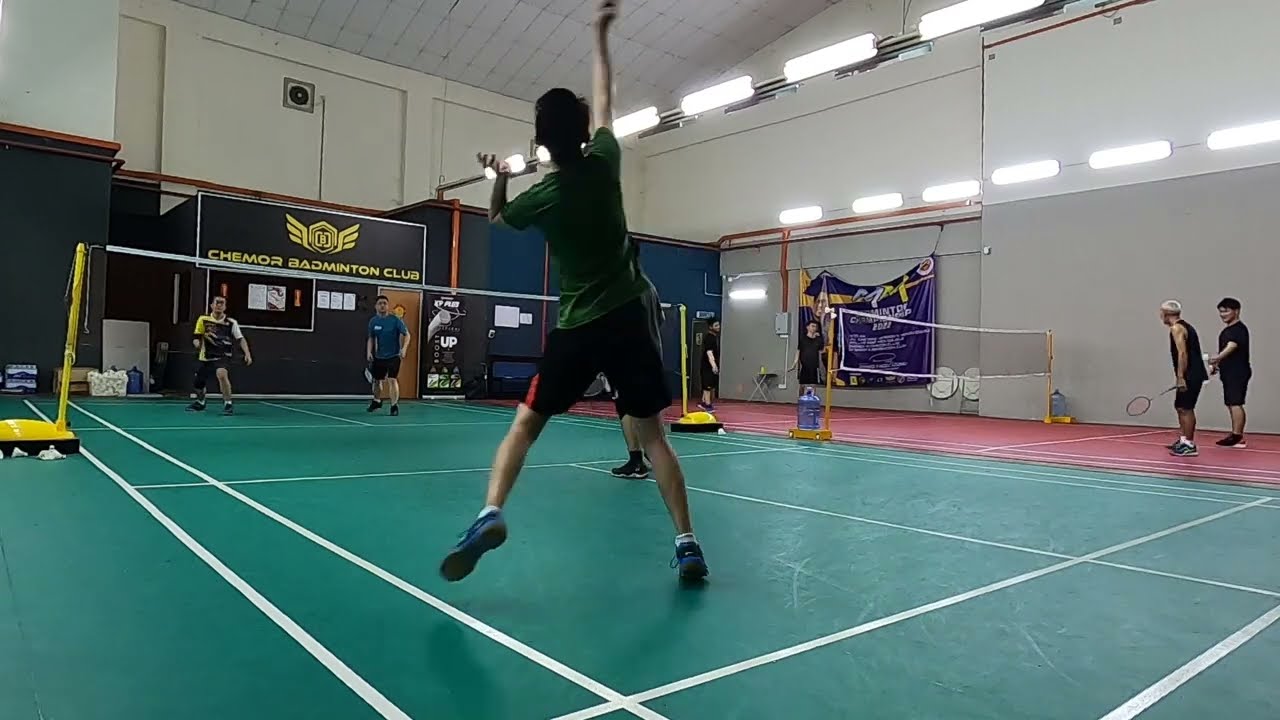The indoor scene captures a bustling environment in the Keymore Badminton Club, featuring two vividly colored badminton courts—one red and one green. Each court has a net dividing it, and there are four teams engaged in doubles matches, with two players per team wielding rackets. In the foreground, a player appears to be leaping to serve, his back facing us. Surrounding the courts, the walls are mainly white with sections painted blue, creating a vibrant backdrop. Above the green court, a sign reading "Keymore Badminton Club" is prominently displayed alongside a logo featuring a flying bee, all done in gold. The words "Cheer More" are also visible, encouraging a lively, spirited atmosphere in the club.